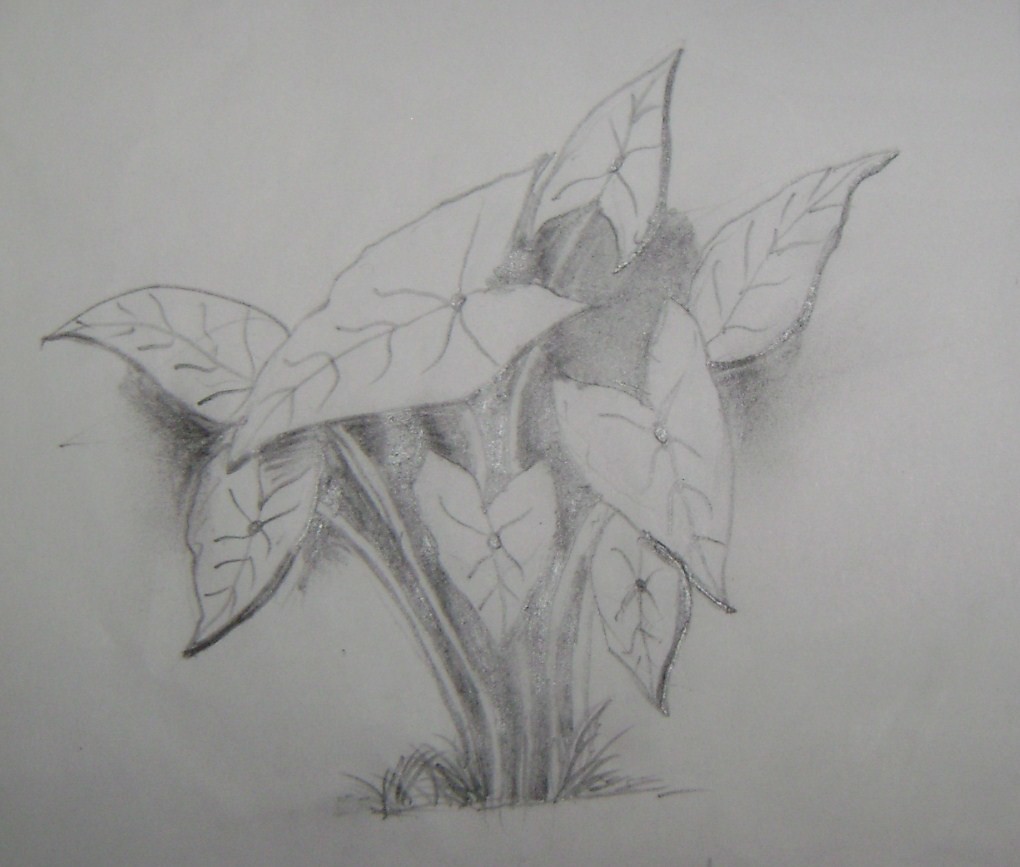The image showcases a meticulously detailed sketch on white paper, dominated by an intricate interplay of pencil marks and varying degrees of light gray shading. The composition features a base of grass at the bottom, with an artful arrangement of leaves sprouting from branches that extend across various parts of the drawing: the upper left, middle left, upper right, and lower right corners. Inside this organic framework, there are numerous fine lines and dots, creating a textured appearance. The intense application of the pencil in certain areas results in a subtle reflection, giving parts of the drawing a metallic silver or very dark gray sheen. This effect adds depth and dimension, making the sketch appear almost three-dimensional.